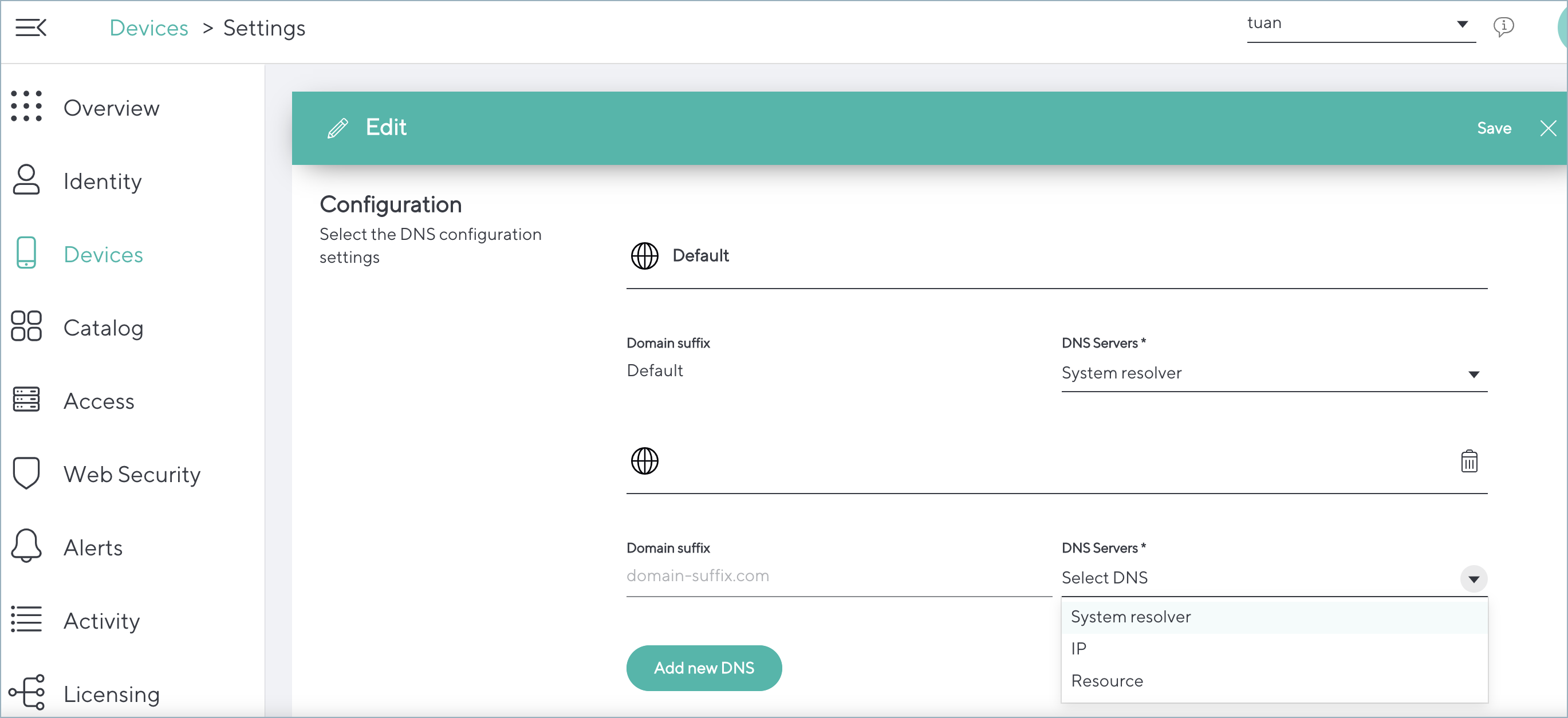Detailed Caption: 

The image is a snapshot of a computer screen displaying a settings page under the "Devices" section. The left-hand side of the interface features a vertical column of icons paired with descriptive labels. Starting from the top, the interface shows:

1. **Overview**: Represented by an icon with nine dots arranged in three rows.
2. **Identity**: Marked by a silhouette of a human figure.
3. **Devices**: Indicated by a cell phone icon and highlighted in green, signifying the active selection.
4. **Catalog**: Shown with four overlapping circles.
5. **Access**: Represented by a rectangle.
6. **Web Security**: Denoted by a shield icon.
7. **Alerts**: Illustrated with a bell.
8. **Activity**: Signified by horizontal lines.
9. **Licensing**: Depicted with a family tree icon.
   
In the main selection area, under the "Devices" tab, a light greenish-blue section labeled "Edit" is visible, featuring a pencil icon next to "Configuration." Below this, there is a "Default" area and a clickable "Add New DNS" button, also in a greenish-blue shade.

This detailed visual layout effectively organizes the various configuration options available on the page.